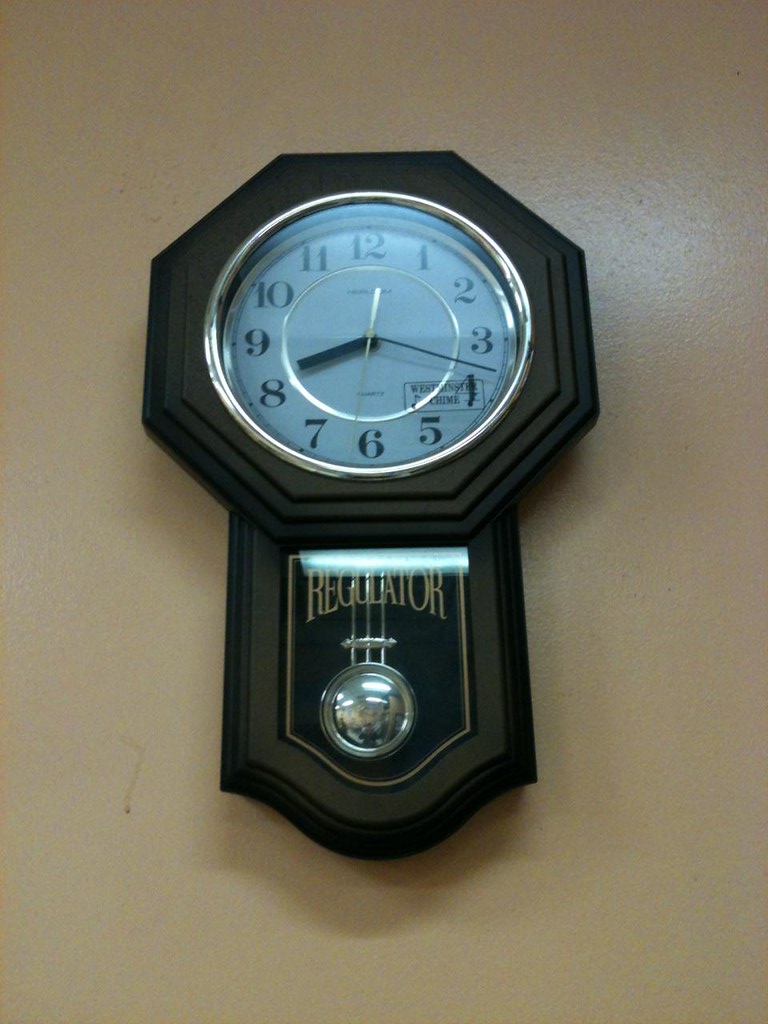This photograph features an intricately designed wall clock, prominently displayed on a subtly textured beige wall. The clock's top portion is framed in an eight-sided hexagonal black shape, accentuating a round, white clock face encircled by a sleek silver ring. The clock face showcases large black numerals, complemented by black hour and minute hands, while the second hand is rendered in a contrasting silver hue. A shiny metal ring subtly decorates the center of the clock face, adding a touch of elegance. Below the clock face, the design transitions into a rectangular extension with a gently curved bottom, incorporating a glass window through which a substantial round silver pendulum is visibly swinging. The word "Regulator" is emblazoned in golden text across this glass window, enhancing its traditional aesthetic. Additionally, a small sticker can be seen in the lower right corner of the clock face's glass covering. This vertical rectangular image captures the timeless beauty and meticulous craftsmanship of the wall clock, making it a captivating focal point.